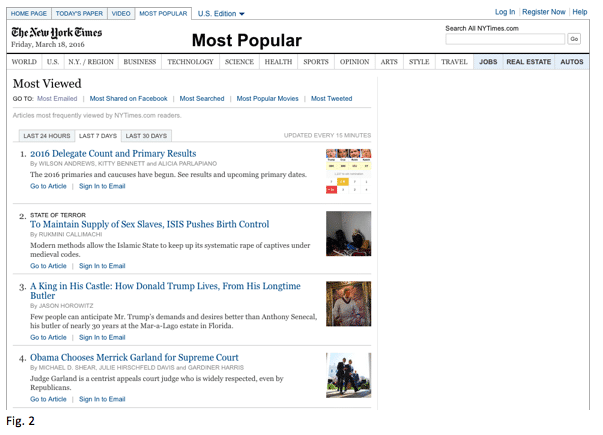This is a detailed and cleaned-up caption for the image described:

---

Screenshot of The New York Times website homepage dated Friday, March 18, 2016. At the top left corner of the webpage, a series of navigation tabs are visible, including "Homepage," "Today's Paper," "Video," and "Most Popular," with the latter being selected. Adjacent to this on the right is a dropdown arrow labelled "U.S. Election" and buttons for "Help," "Register Now," and "Log In" are found in the upper right-hand corner.

Centered at the top of the page, the iconic "The New York Times" logo is prominently displayed with the date directly below it. A search bar labelled "Search All NYTimes.com" with an accompanying "Go" button is situated on the top right side. Just beneath, various sections of the newspaper are listed in a horizontal menu, including "World," "U.S.," "N.Y.-Region," "Business," "Technology," "Science," "Health," "Sports," "Opinion," "Arts," "Style," "Travel," "Jobs," "Real Estate," and "Autos."

Further down the page, categorized sections such as "Most Viewed," "Most Emailed," "Most Shared on Facebook," "Most Searched," and "Most Tweeted" are positioned above another search bar that reads "Articles Most Frequently Viewed by NYTimes.com Readers." Below this search bar, four clickable article links are displayed under a tab labelled "Last 7 Days."

---

This caption provides a comprehensive and visually informative description of the image, ensuring clarity and detail about the webpage's layout and content.